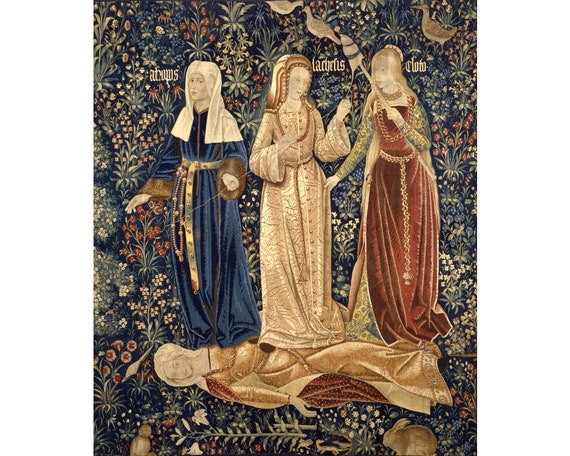This image is an intricate drawing depicting four women against an ornate, medieval-like background filled with floral designs and various birds. The background, reminiscent of vintage wallpaper, features sprigs of flowers in shades of white, red, pink, and green, along with images of ducks, a bird sitting on the bottom left, and a rabbit on the bottom right.

The women are named Alanis, Ladris, and Colin, with one figure remaining unnamed. The unnamed woman lies on the floor in tan robes. The other three women are standing over her, each adorned in distinct attire: one in a blue robe with a gold belt, beads, and a white towel over her head; the central figure in a gold brocade gown fastened from neck to feet, with a rope tie; and the third woman in a reddish-brown, velvet-like dress holding a stick with a bird perched on it. Two of these upright women wear ornate headpieces, adding to the scene's elaborate and historical aesthetic.